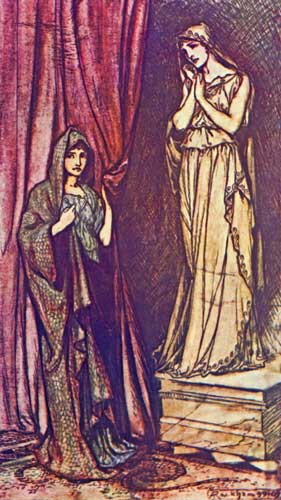In this detailed, hand-painted illustration set in a classical, possibly Greco-Roman, historical setting, a woman in a pink dress layered with a red shawl stands in the bottom left corner of the image. She clutches a red curtain that extends floor to ceiling, with visible pleats and gathers, forming a striking backdrop. The ornate ground beneath her appears to be an intricate tile or rug patterned in red tones. Facing right, she directs her gaze towards a statue positioned in the top right. The statue, carved in light colors, depicts a woman in long Greek-style robes and a hooded cloak, mirroring the clothing of the living woman. The statue's arms are bare and arranged such that her palms are held together, moving upwards towards her chin, conveying a compassionate expression. The overall composition suggests a careful alignment of the living figure and the statue, emphasizing their visual and thematic similarities. The entire scene is imbued with hues of red, brown, gray, tan, yellow, and green, capturing a rich, historical ambiance without any text to distract from its classical beauty.